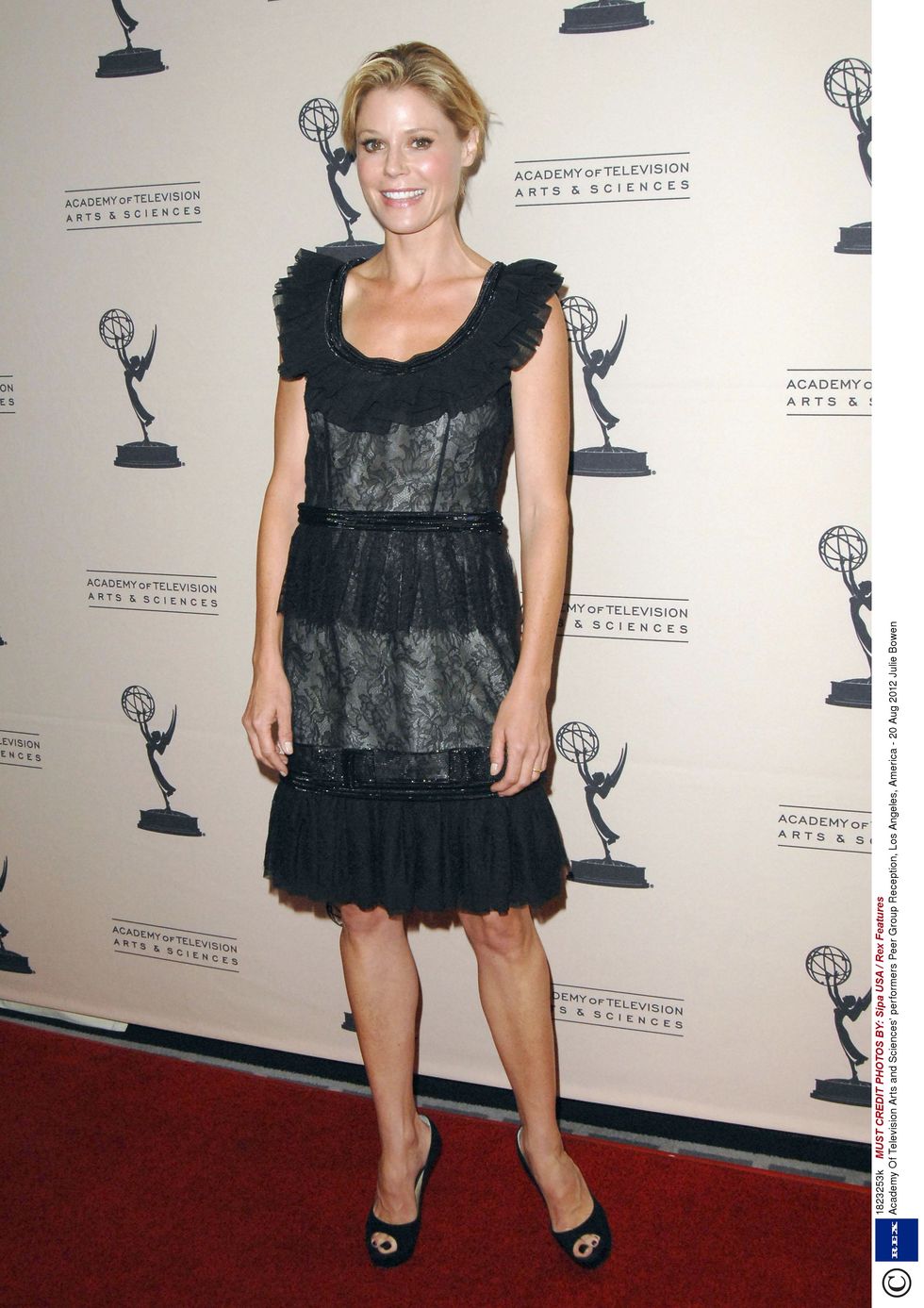In this image, we see a woman standing on a red carpet at an event hosted by the Academy of Television Arts and Sciences. The backdrop features a repeating pattern of the Academy's logo, which is a winged figure holding a globe, and the text "Academy of Television Arts and Sciences" printed prominently in multiple rows. The woman, identified as Julie Bowen, is smiling brightly at the camera. She has her blonde hair pulled back, showcasing her light brown eyes. She is dressed in a sleeveless black dress adorned with frills around the neckline, waist, and hem. Her outfit is complemented by black, open-toed high-heel sandals, and her toenails are painted black. To the right of the image, there is copyright information that includes the phrases, "must credit photos by SIPAUSH / REX Pictures," and details about the event, which took place on August 20, 2012, in Los Angeles.